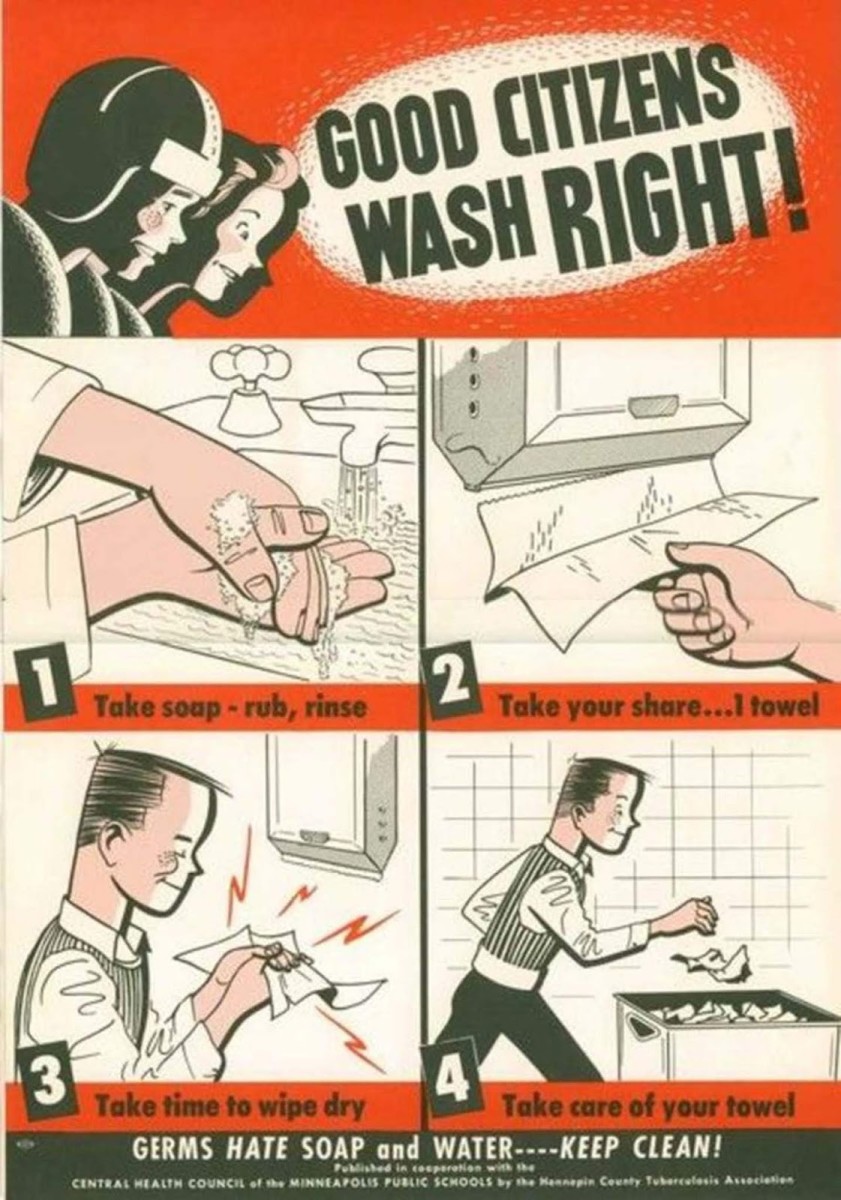This detailed health poster, titled "GOOD CITIZENS WASH RIGHT!", provides illustrated instructions on proper hand hygiene. The poster features a red background with two characters, a woman and a man, looking downwards towards the steps. The title is prominently displayed in all caps within a white oval, encased in a black border. 

The instructional content is divided into four steps, each accompanied by corresponding hand-drawn illustrations:
1. **Take Soap, Rub, Rinse:** Depicts hands lathering soap under running water.
2. **Take Your Share, One Towel:** Shows a hand grabbing a single paper towel from a dispenser.
3. **Take Time to Wipe Dry:** Illustrates a person drying their hands with the paper towel.
4. **Take Care of Your Towel:** Features an individual disposing of the used paper towel into a trash bin.

At the bottom of the poster, a black text box with a white font states, "GERMS HATE SOAP AND WATER - KEEP CLEAN." Additionally, there is small, unreadable text attributed to cooperation with the General Health Council of the Minneapolis Public Schools and the Something County Tuberculosis Association.